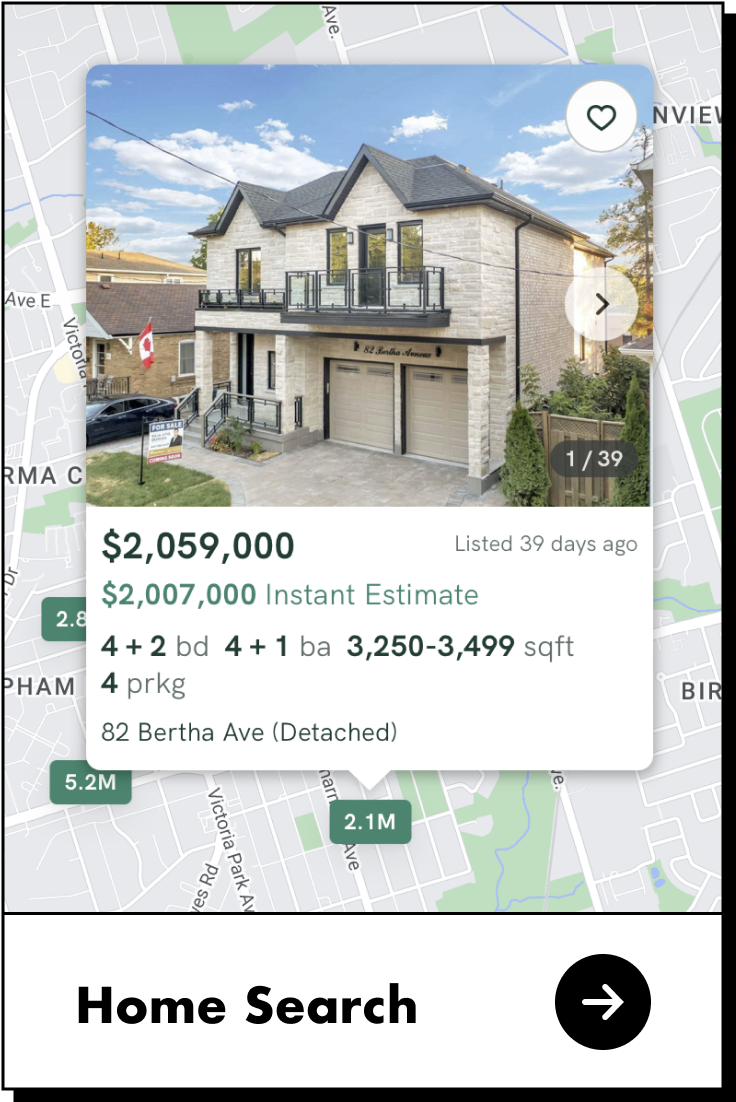This image showcases a detailed screenshot from a home search on a smartphone, highlighting a house listed for sale. At the bottom of the screen, there's a "Home Search" label displayed in black text on a white rectangle, accompanied by a right-pointing white arrow within a black circle. The top features a clear picture of a two-story detached house, characterized by two prominent gable peaks above the windows. The house includes two garage parking spaces and what appears to be a sophisticated driveway. Notably, a Canadian flag is visible near the front of the house.

Further information indicates there are a total of 39 images available for viewing. The house is priced at $2,059,000 with an instant estimate valuation of $2,007,000. It offers spacious accommodation with four plus two bedrooms and four plus one bathrooms. The living area measures between 3,250 to 3,499 square feet. Additionally, the listing notes that there are four parking spaces available. The property is located at 82 Bertha Avenue.